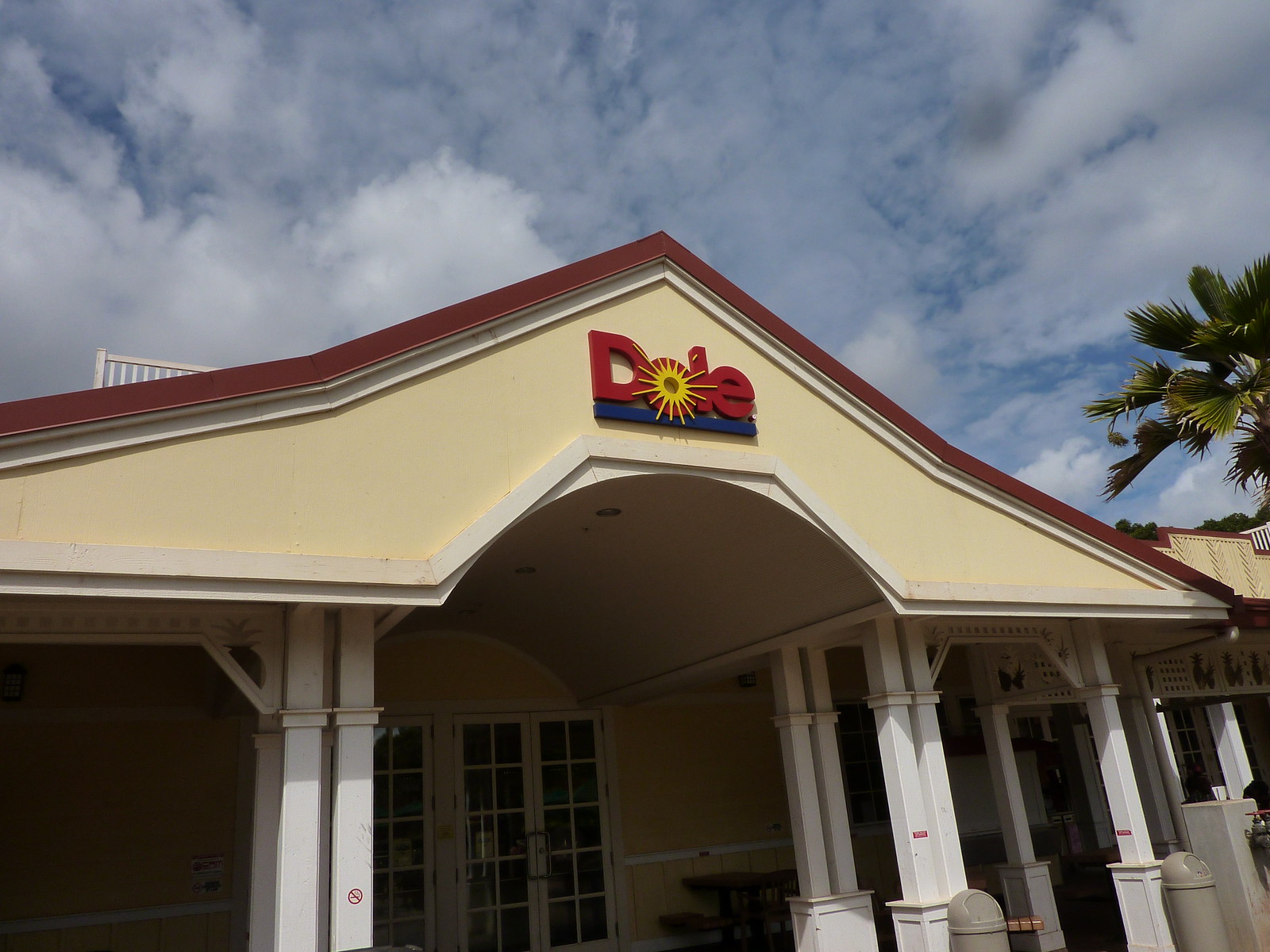The photograph captures the front facade of an outdoor building on a sunny day. Against a backdrop of a vivid blue sky peppered with fluffy white clouds, the structure is prominently featured. The building boasts a stately design, characterized by columns at its entrance and a peaked, dark brown roof. The side of the roof facing the camera is painted in a creamy yellow hue, creating a pleasing contrast with the brown. Above an archway, the vibrant Dole logo stands out, with its bold red letters and a cheerful yellow sun incorporated into the "O," all underlined by a striking dark blue line. The top edge of a palm tree is visible to the right, adding a touch of tropical charm to the scene.